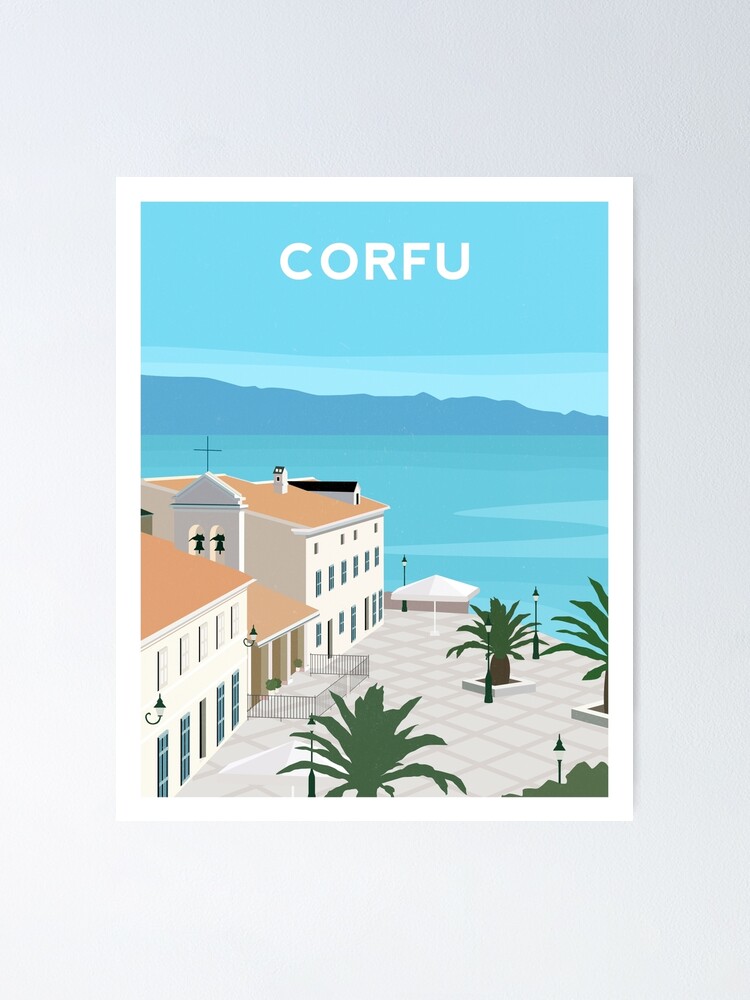This artwork, possibly a computer-generated or animated poster, hangs on a light gray wall and features a white outer border. At the top of the image, in white capital letters, is the word "CORFU." The sky above exhibits various shades of light blue, transitioning into a blue-violet mountain range. Below, there are two differently shaded blue waters.

The central focus is a series of hand-drawn buildings with cream-colored facades and pale salmon roofs. Among them, a prominent church stands out with a white steeple, a cross, and two black bells hanging within a tower. Dark gray windows punctuate the buildings, indicating they might be part of a hotel or business complex within a resort area. 

In front of these structures lies a large patio area with neatly sectioned white tile flooring and a variety of elements such as a white umbrella, a streetlight, and several lamp posts. Additionally, four green, tropical-looking trees, perhaps in planter-like white squares, are strategically positioned around the space. A black metal gate marks the entrance, enhancing the overall tropical resort vibe.